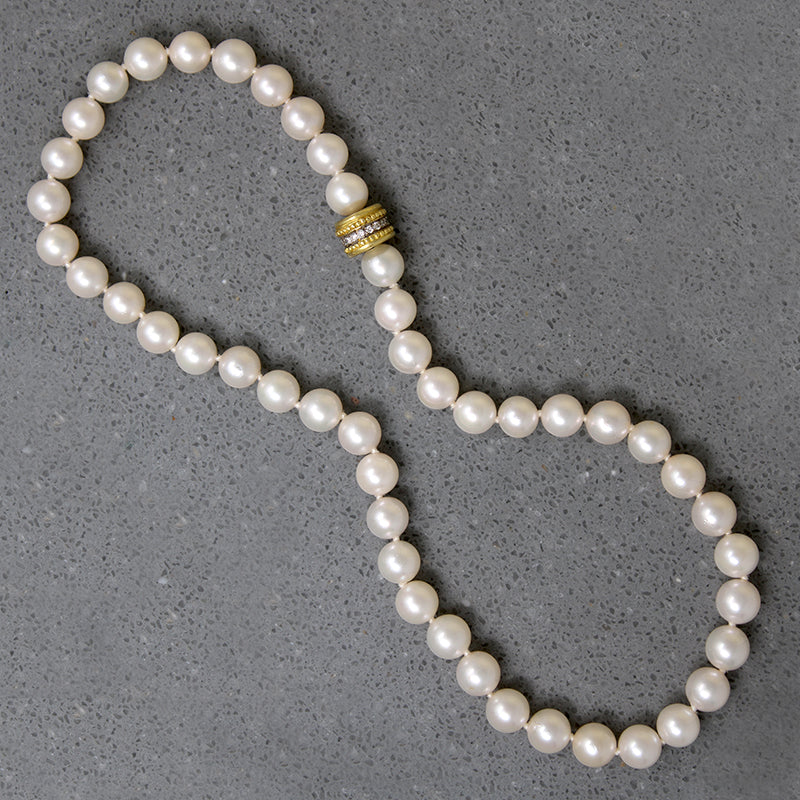The image features a small yet intricately designed pearl necklace displayed on a gray, granite-like background. The luminous white pearls are uniformly circular and range from half an inch to an inch in diameter. They are strung together meticulously, showing a consistent color and subtle iridescence. The centerpiece of the necklace is a striking gold bead positioned precisely in the middle, adorned with shiny diamonds along its center. This bead is flanked by gold clasps, adding to the necklace's elegance and hinting at its high value. The necklace is artfully arranged in an oval pattern, reminiscent of a peanut shell or the number eight, where the center narrows before expanding back into a broader curve at each end. The careful placement and exquisite craftsmanship suggest high-quality materials and a refined aesthetic.